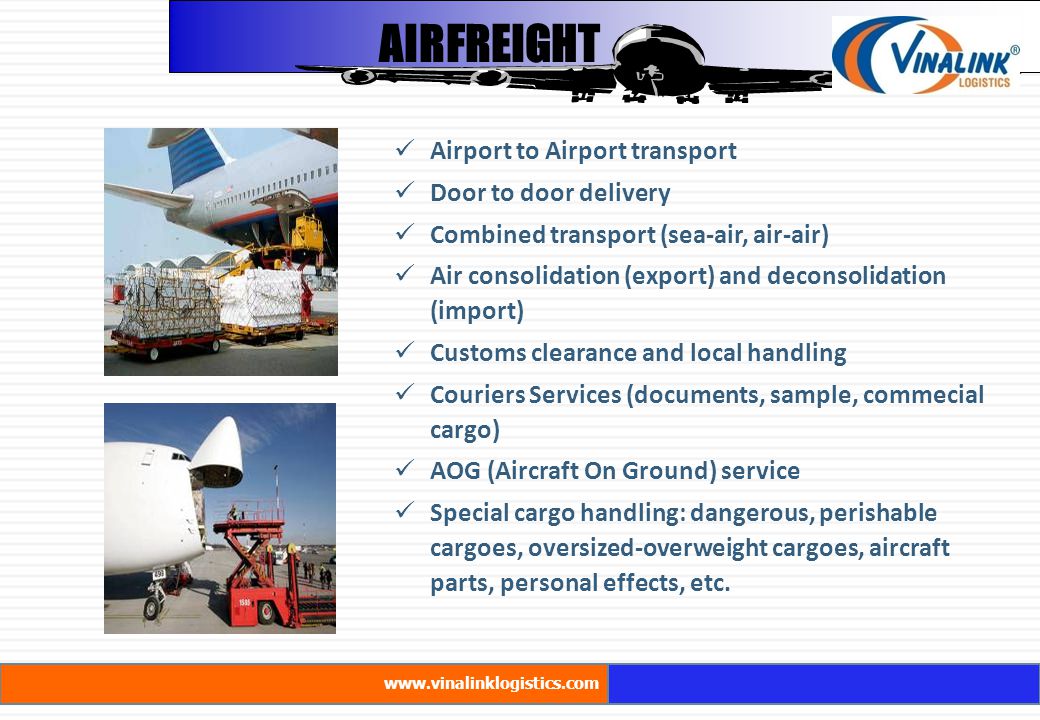The image depicts a web page for Vinna Link Logistics, highlighting their air freight services. At the top, the words "Air Freight" are prominently displayed next to a black and white airplane graphic. To the right, the logo "Vinna Link Logistics" is visible. Below this, the detailed text against a lined white background lists extensive services: airport to airport transport, door-to-door delivery, combined transport, sea-air and air-air options, air consolidation and deconsolidation, customs clearance, local handling, courier services, AOG (Aircraft on Ground) service, special cargo handling, and provisions for dangerous, perishable, oversized, and overweight cargos, including aircraft parts and personal effects.

On the left side of the page, there are two images. The top image shows cargo being loaded into the back of a white airplane with a blue fin and underbelly, set against an airport tarmac with red and yellow markers. The bottom image features a plane with its nose open for maintenance, with visible equipment and personnel in the background, set under a blue sky. At the bottom of the page, an orange box next to a blue box displays the website address: www.vinnalinklogistics.com.